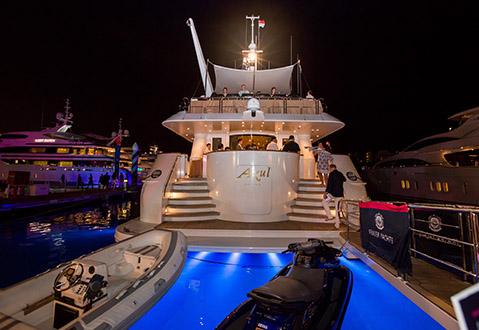This image captures a nighttime view of a luxurious yacht party. The party is taking place on a multi-deck white yacht docked alongside another yacht and what seems to be a nearby building, possibly a restaurant. The backdrop is an inky black sky, enhancing the brilliant blue illumination of the yacht's pool on the lower deck, which also contains a small lifeboat and a black jet ski.

We are looking at the yacht from the rear, where attendees are seen walking up a set of wide stairs bordered by handrails, leading to the main deck. This middle deck is bathed in warm golden light and bustling with people, indicating the main site of the festivities. The yacht's railing on the right side displays a black and red banner adorned with a white logo.

Above the main deck, an upper floor sheltered by a canopy holds additional guests, who are visible through the glow from overhead lighting. Overall, the scene exudes opulence and festivity, capturing a vibrant social gathering under the night sky, reflecting in the blue-water lights.